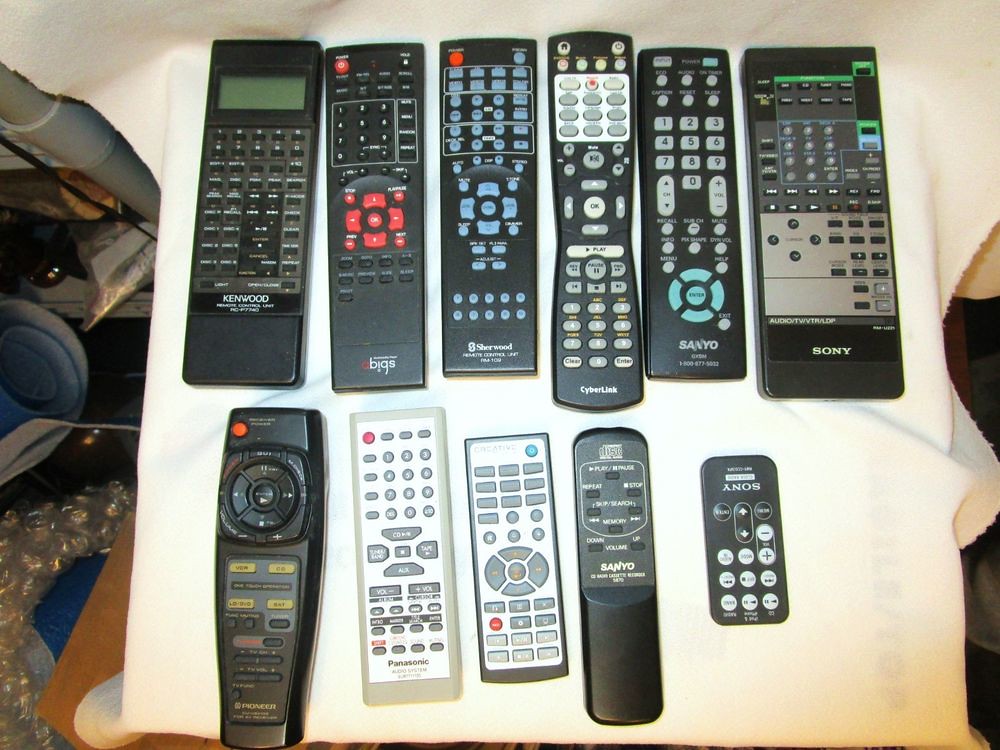This detailed photograph captures an assortment of 11 remote controls of varying sizes and styles, arranged on what appears to be a white piece of cloth or towel draped over a flat surface. The majority of these remotes are black, except for a prominent white Panasonic model at the bottom. The remotes showcase a diverse range of brands, including Sony, Sanyo, Sherwood, CyberLink, Pioneer, Kenwood, and Creative. Several remotes feature complex button layouts, with most containing around 25 to 40 buttons, while a few, like the inverted Sony remote, have fewer buttons in a more simplified design. One remote is distinguished by an LCD display, though it is not currently active. The remotes feature buttons in multiple colors—blue, red, white, and black—adding visual interest. Notably, one remote has a radial button arrangement with a central button surrounded by four outer buttons. Surrounding the crisp white cloth are some miscellaneous items scattered on the floor, adding a casual, everyday context to the scene.